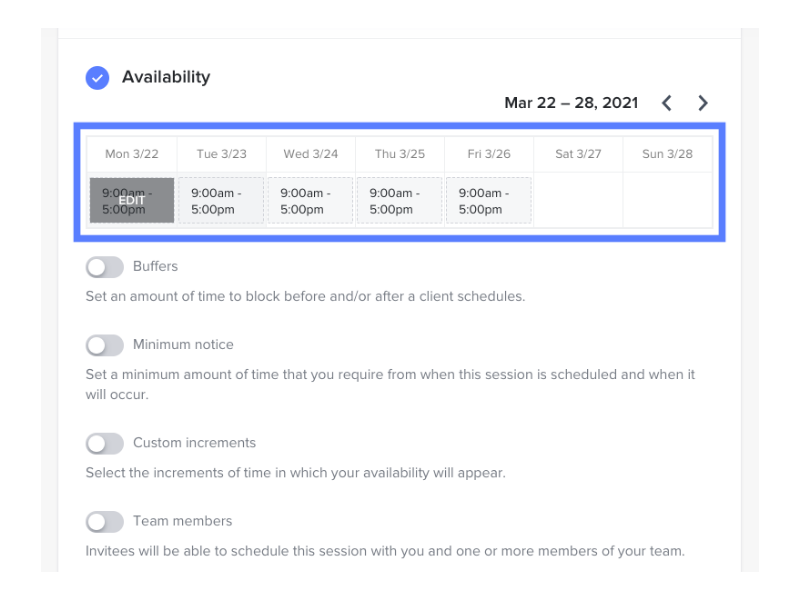A screenshot of a scheduling app with a clean, user-friendly interface on a white background. In the top left corner, there's a blue circle featuring a white check mark, labeled "Availability." Just below and to the right, a selected time frame is displayed, reading "March 22nd to the 28th 2021," flanked by back and forward navigation arrows.

Underneath, a weekly calendar is presented for the specified time frame, highlighted with a blue border that encompasses the dates. Each day from Monday (3/22) to Friday (3/26) is listed with the working hours of 9 a.m. to 5 p.m. Notably, Monday (3/22) also has a gray "Edit" button with white text, allowing for modifications. Weekend dates, Saturday (3/27) and Sunday (3/28), show no scheduled entries.

Beneath the calendar, there are four distinct toggle switches, all in the 'off' position:
1. **Buffer** - Allows setting a block of time before and/or after a client schedules.
2. **Minimum Notice** - Sets the minimum time required between scheduling a session and its occurrence.
3. **Custom Increments** - Allows selection of time increments for availability.
4. **Team Members** - Lets invitees schedule the session with you and one or more team members.